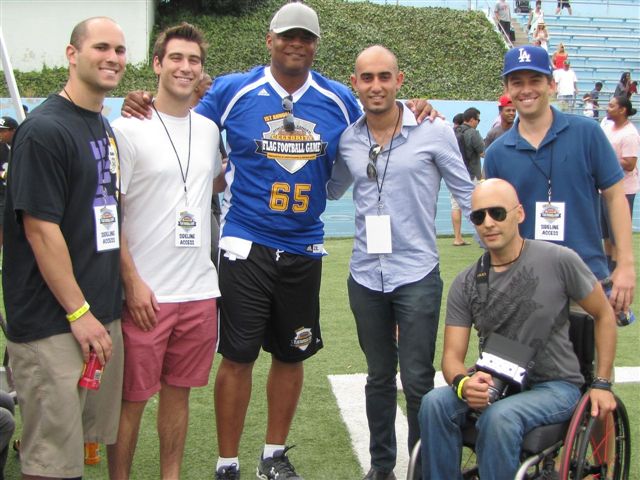In an outdoor, sports-field setting, the image features six men prominently positioned at the forefront. From left to right:

- The first is a white male with shaved brown hair, wearing a black t-shirt with purple writing and beige shorts.
- Next to him stands another white male with styled hair, donning a white short-sleeved t-shirt and pink shorts.
- The third, a black male, sports a blue "Flag Football Game" top, a white cap, and black shorts.
- The fourth male, possibly white, has a shaved head, a light blue shirt with sunglasses tucked in, and dark-colored trousers.
- The fifth has on a blue polo shirt, a blue cap with "LA", and stands behind the sixth man, who is in a wheelchair.
- The man in the wheelchair, bald and wearing sunglasses, has a gray top and blue jeans and stands in front of the fifth man.

All but the man in the wheelchair are smiling. Behind them, on the right, there are blue bleacher stands filled with people, raised seating, and a bluish track surface. The men stand on a grassy sports field, indicated by visible white markings on the grass, and additional people can be seen in the background on a grassy incline.